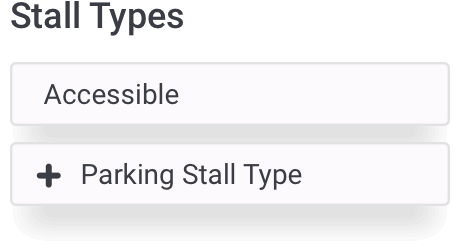This small, straightforward image features minimal information, presented with meticulous attention to detail. Dominating the top of the image is a prominent title in large black text: "STALL TYPES." Below this heading, two distinct options are displayed, each enclosed within a white rectangle outlined in light grey, giving them a subtle 3D effect through light to medium grey shadows.

The first rectangle centers the word "accessible" in black text, clearly indicating the type of stall. Directly beneath this, the second rectangle contains a bold, dark plus sign symbol. To the right of this symbol, written in black text, are the words "parking stall type."

The consistent use of black text for all verbal elements contrasts sharply with the white background of the rectangles, ensuring clear readability. The light grey outlines and the shadow effect beneath each rectangle add a touch of depth, making the elements appear as though they are gently hovering off the page.